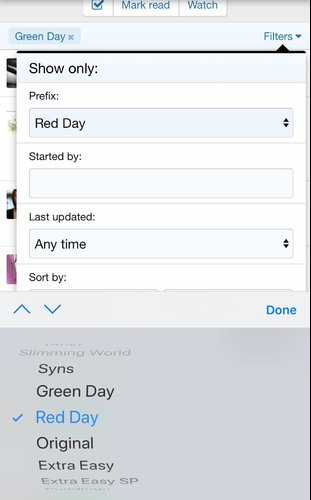The image appears to be a partial screenshot of an application interface, possibly for a mobile device or webpage. At the top of the screen, there is a partially cut-off section featuring a checkmark icon followed by the text "Mark Read" or "Watch." Below this, the image prominently displays the name "Green Day," which could refer to the band but is not entirely certain in this context.

To the right of "Green Day," there is a "Filters" option. The central part of the image contains a large black-font heading that says "Show Only," followed by the word "Prefix" and a dropdown menu currently set to "Red Day." 

Further down, there is a section labeled "Started By," which has an empty selection box next to it. Below that, the terms "Last Updated" appear, with a dropdown set to "Any Time." Following this, there is a "Sort By" option leading to the term "Done."

In the lower part of the screen, there appears to be a rolling selection menu, with the first and last options slightly blurred out, indicating a scrolling effect. Visible options in this rolling menu include "Sins," "Green Day," "Red Day," "Original," and "Extra Easy." This suggests the screen is part of a user interface for selecting various options, possibly for an application or game, where selections such as "Green Day" and "Red Day" are available choices.